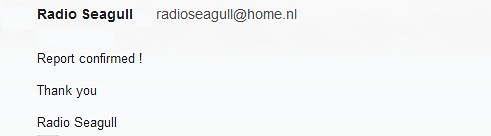The rectangular image, approximately three inches wide and one inch tall, features a very faint grayish-blue or slightly off-white background, with no visible border. In the top left corner, there is bold black text that reads "Radio Siegel." Just to the right of this bold text, in smaller, unbolded black font, it reads "RadioSiegel@home.nl," the email address associated with the Netherlands domain. Beneath this and slightly lower, it says "Report Confirmed!" in small black print, followed by "Thank You." Towards the bottom of the rectangle, the text repeats "Radio Siegel," maintaining consistency in black, unbolded font. The entire graphic provides a confirmation or verification message, likely resembling an email format.